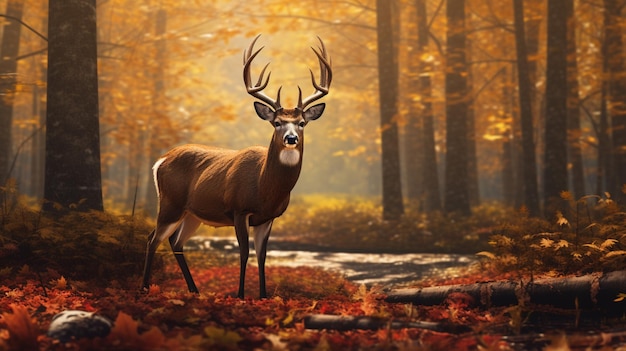In this vibrant and possibly AI-generated surreal image, a majestic buck stands prominently in a well-lit autumn forest. The deer, with its brown coat and distinct white circles under its mouth, gazes directly at the viewer. It boasts an impressive set of twelve-point antlers, whose spiky branches reach towards the center. The buck's legs are black near its feet and turn white near the torso. Surrounding the deer, the forest floor is a tapestry of red and amber leaves. Behind the buck, a small stream weaves through a landscape interspersed with fallen logs and rocks. Tall, thin tree trunks rise up from the ground, their tops disappearing out of the frame. The sunlight, either from a sunrise or sunset, breaks through the forest canopy, casting a golden hue across the scene and illuminating the vibrant leaves, amplifying the surreal, almost unrealistic beauty of the image.